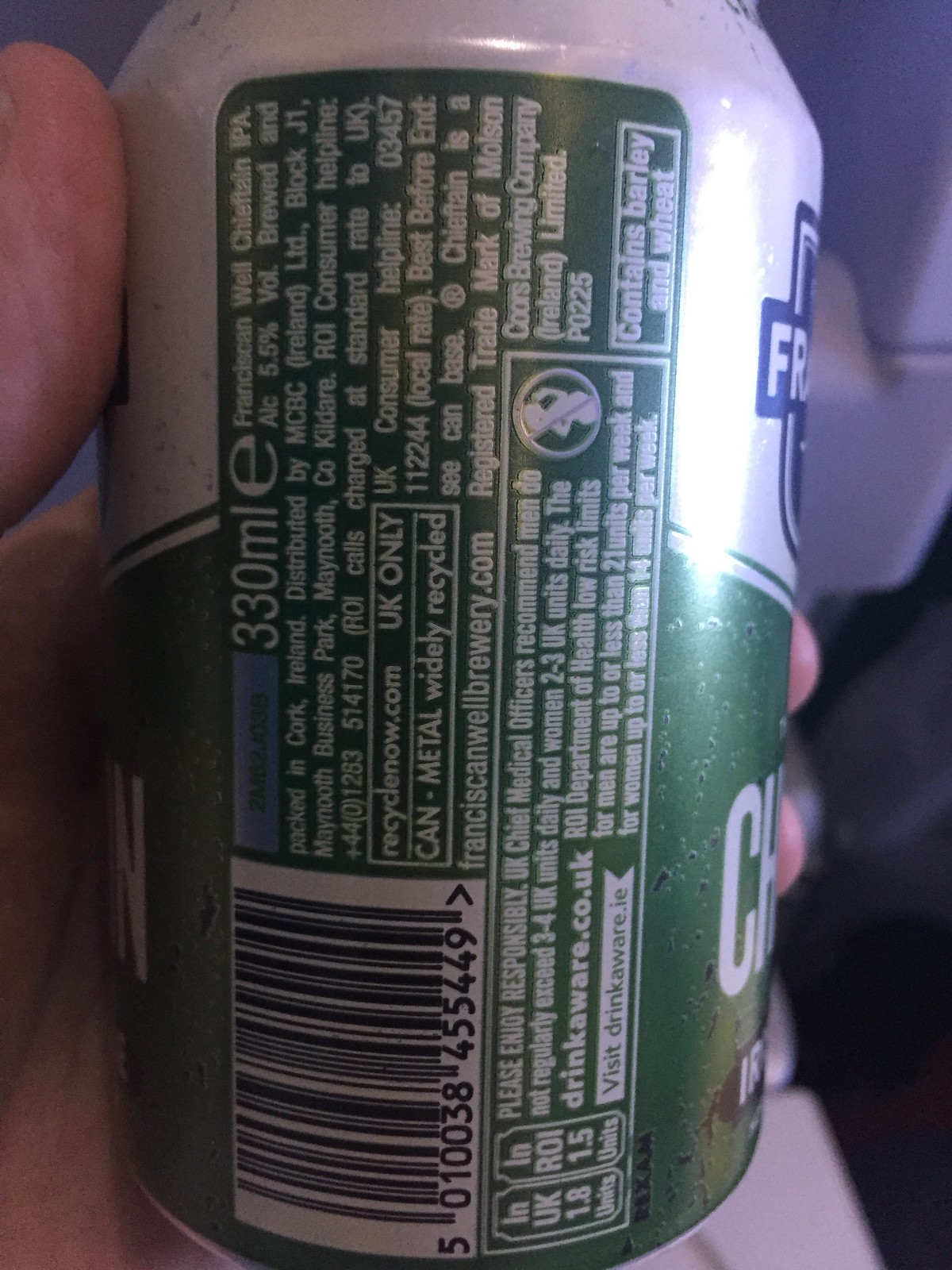A close-up image captures a hand, likely male, holding a silver and dark green can. The visible portion of the hand includes the thumb, fingertips, and part of the palm, without any visible nails. The can is positioned to display its nutritional facts label prominently. The upper half of the can is silver, while the lower half is dark green. A large blue logo with white lettering is partially visible on the front of the can. The background is blurred, with indistinct objects adding to the focus on the hand and can.